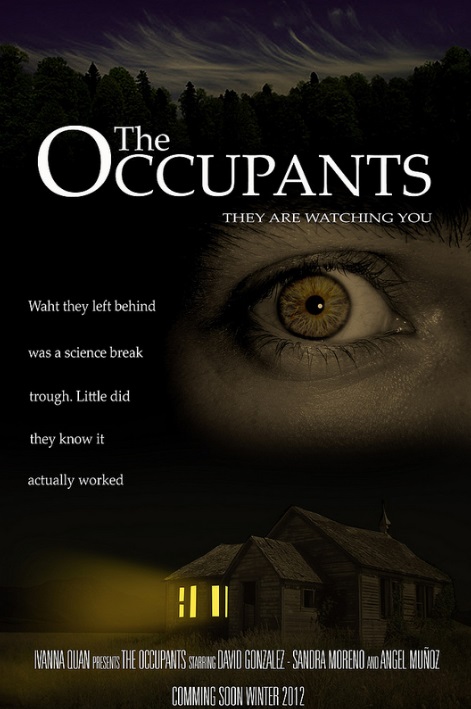The movie poster for "The Occupants" is captivating and eerie, drawing immediate attention with a close-up of a wide-open light blue eye that appears to be watching you. The eye, which seems to belong to a woman, is prominently featured at the top of the poster against a dark backdrop. Beneath the eye, an ominous image of a wooden house bathed in darkness appears, with a single yellow-lit window providing a stark contrast. The house looks unsettling, situated against a night sky with silhouetted trees adding to the sinister mood. The title "The Occupants" is boldly displayed in large white font, and a chilling tagline reads, "They are watching you." Another tagline to the left states, "What they left behind was a science breakthrough. Little did they know it actually worked." The names Ivana Quan presents, alongside David Gonzalez, Sandra Moreno, and Angel Munoz, are listed as the featured actors. At the bottom, the poster notes that the movie is coming soon in winter 2012. Despite some minor spelling errors, the design effectively sets a creepy tone that intrigues and unsettles.